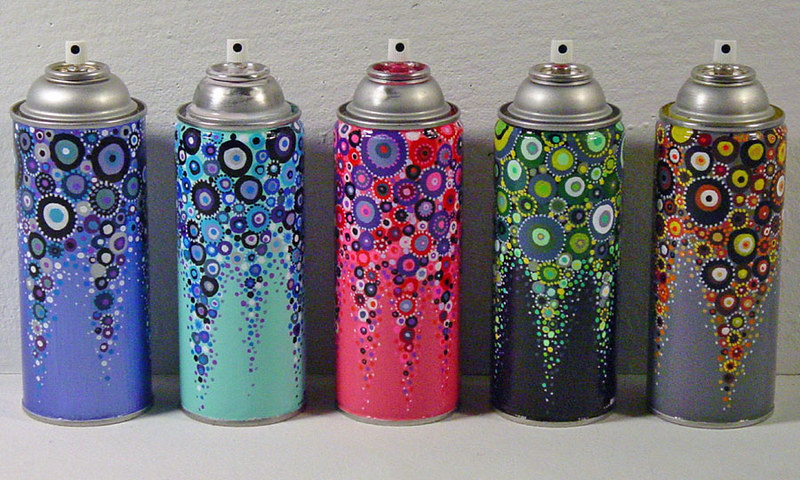This detailed color photograph captures five aerosol spray paint cans, meticulously lined up against a gray wall on a gray surface. All cans have white nozzles with black centers, and lack caps, with their chrome tops prominently facing the camera. Each can features a striking, intricate design that resembles cellular or bubble-like images made up of multicolored circles. From left to right, the sequences of the cans are as follows: the first can has a royal blue base, the second is turquoise, the center can stands out with its pinkish-red hue with a hint of red paint visible, the fourth is dark green, and the fifth can exhibits a primarily gray color. The background of the image is also gray, suggesting the cans are possibly displayed on a gray shelf. The photograph's close-up perspective emphasizes the decorative and chromatic details on each can, enhancing their visual appeal.